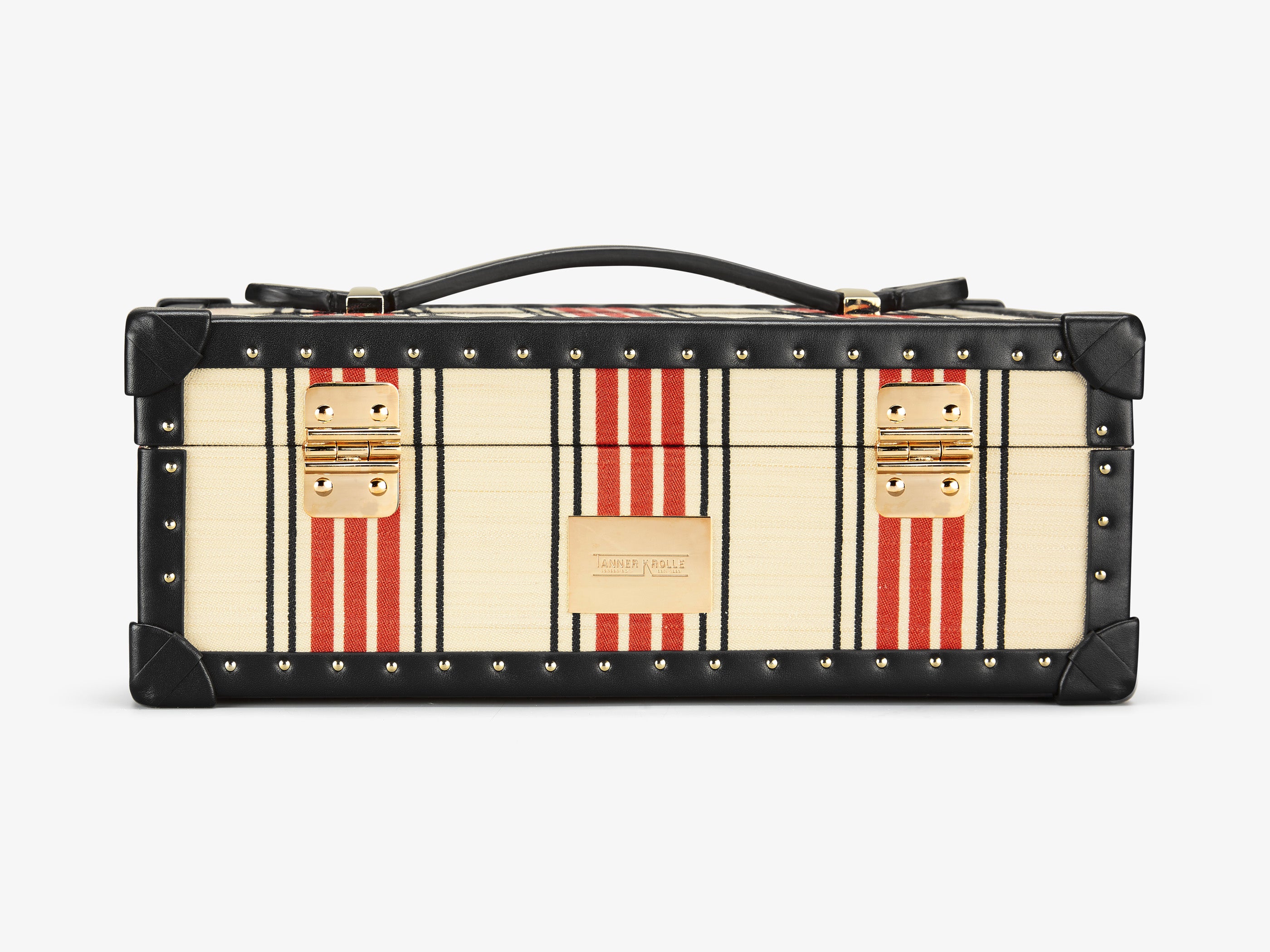This photograph features a vintage-style suitcase displayed against a plain white background. The suitcase, primarily made from a cream-colored canvas-like fabric, is decorated with vertical stripes. The design includes three thick orange/red stripes flanked by thin black stripes, which repeat three times along the length of the suitcase. The borders and edges are meticulously bound in black leather, reinforced with silver metal rivets for added durability. The suitcase has gold-tone hinges at the back and gold brackets securing a black leather handle on top. The front features two robust gold latches, each fastened with four screws. In the center of the suitcase, a tan leather label, although faint and embossed, bears the manufacturer's name, likely "Tanner Roll." The suitcase's overall rectangular shape is accentuated by the leather and metal detailing, giving it a sturdy yet elegant appearance.